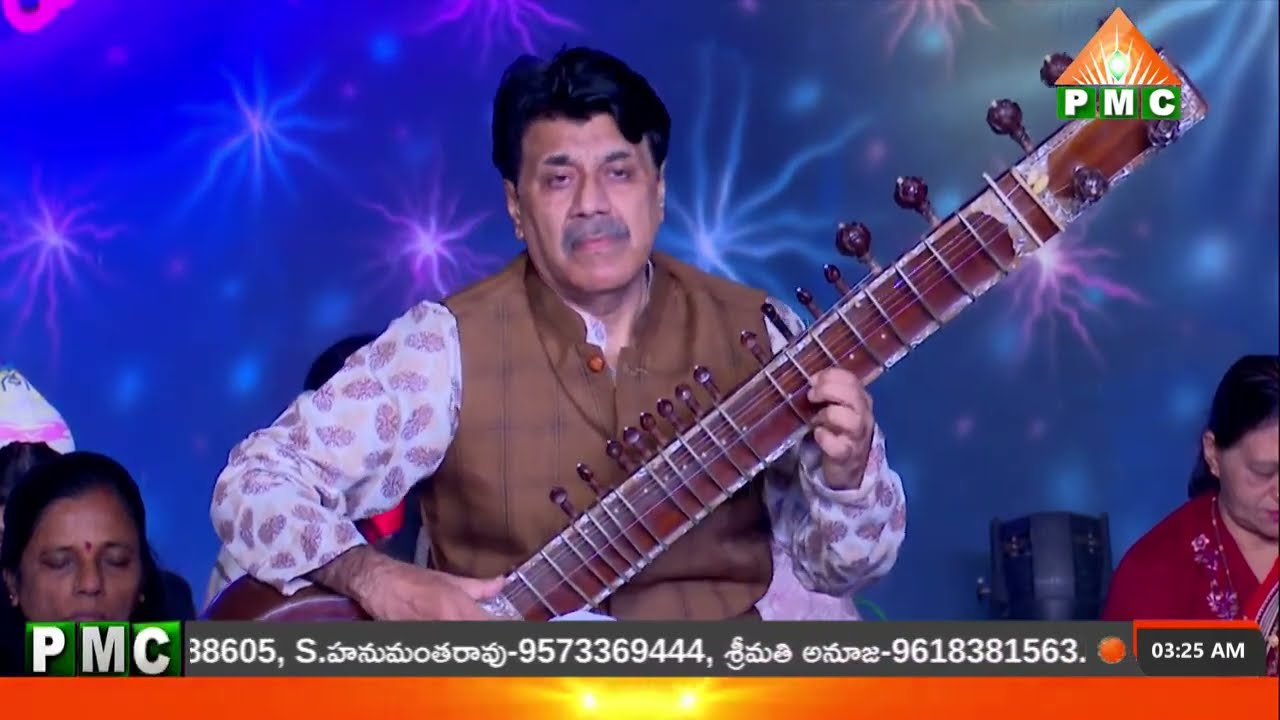The image depicts a serious-faced man with a gray mustache and black hair, wearing a brown vest over a white shirt adorned with leaf-like designs on the sleeves. He is holding a sitar, an Indian string instrument, in his left hand, with its long body featuring circular protrusions extending towards the top right of the image. Behind him, on either side, are two women with closed eyes; the woman on the left has brown hair and a red dot on her forehead, while the woman on the right has black hair and wears a red outfit. The background is blue, and there is a prominent logo in the top right corner comprising a yellow triangle with a diamond inside, labeled PMC. Below it, a gray bar runs across the screen displaying various numbers and symbols, including 38605 and 9618381563, alongside another bar that reads PMC in a white font on a blue background. The bottom of the image features an orange bar punctuated by two bright yellow lights and text that includes the time 3:25 AM.